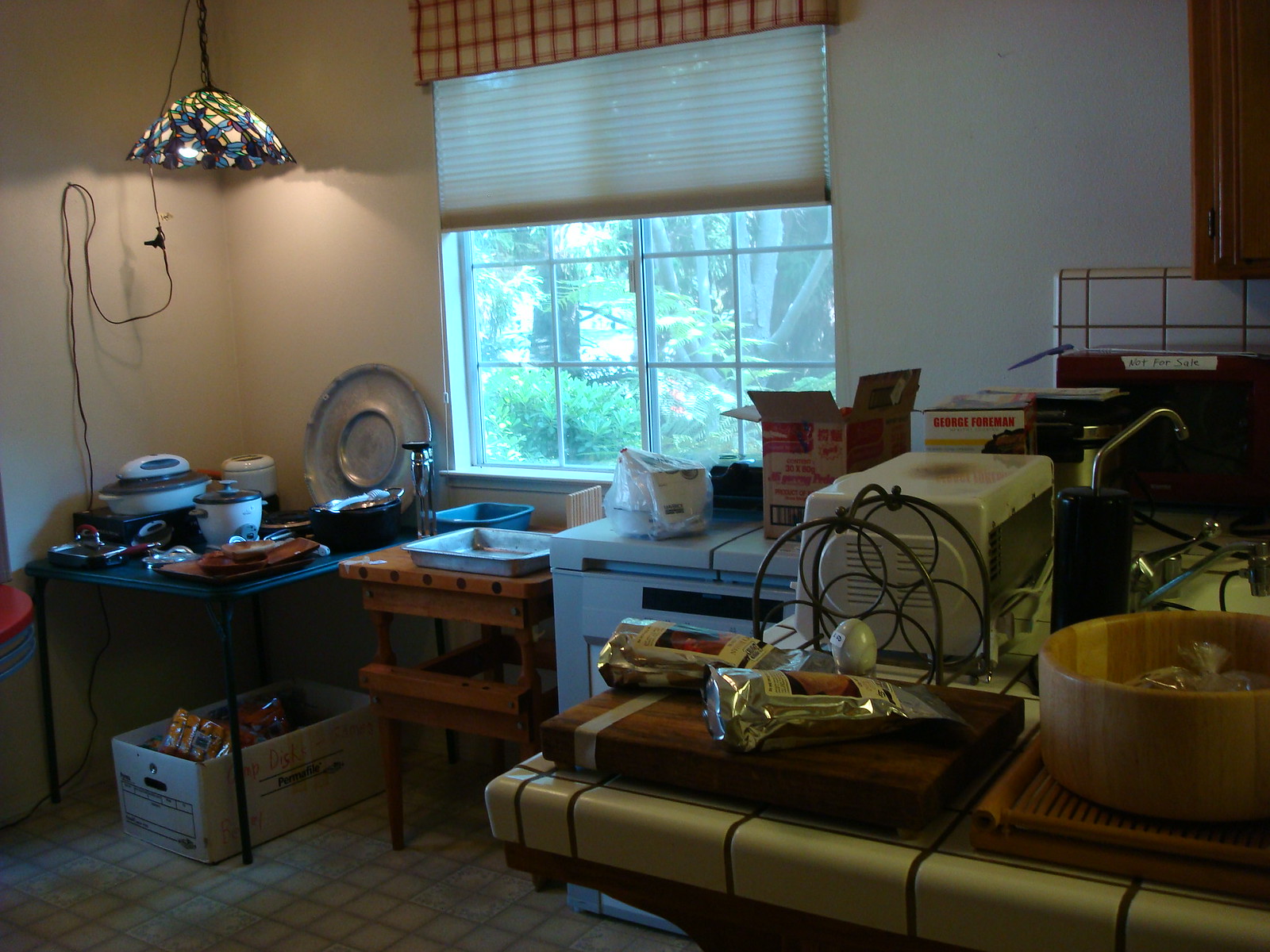The kitchen is brightly illuminated by natural light streaming through a large, paneled sliding window at the center of the room. This window is dressed with a charming red and white valance and a white fold-up shade, allowing a generous amount of sunlight to flood in. Outside, the view reveals lush green trees and vibrant shrubs, enhancing the room’s freshness.

Inside, various surfaces populate the kitchen, showcasing a mix of functionality and temporary storage solutions. In one corner, there is a black pop-up temporary table laden with an assortment of dishes. Below this table, a box filled with groceries and several glossy yellow bags are conveniently stored. 

A striking decorative element in the room is the Tiffany-style glass lamp hanging from the ceiling by a long black cord. Its intricate design features shades of blue, white, and black which add a touch of elegance to the space.

A small brown table nearby supports an aluminum pan, while adjacent to it, a compact white drawer unit appears to house a dishwasher. Across the kitchen, white-tiled surfaces host an array of appliances, contributing to the room's overall utility and organized appearance.